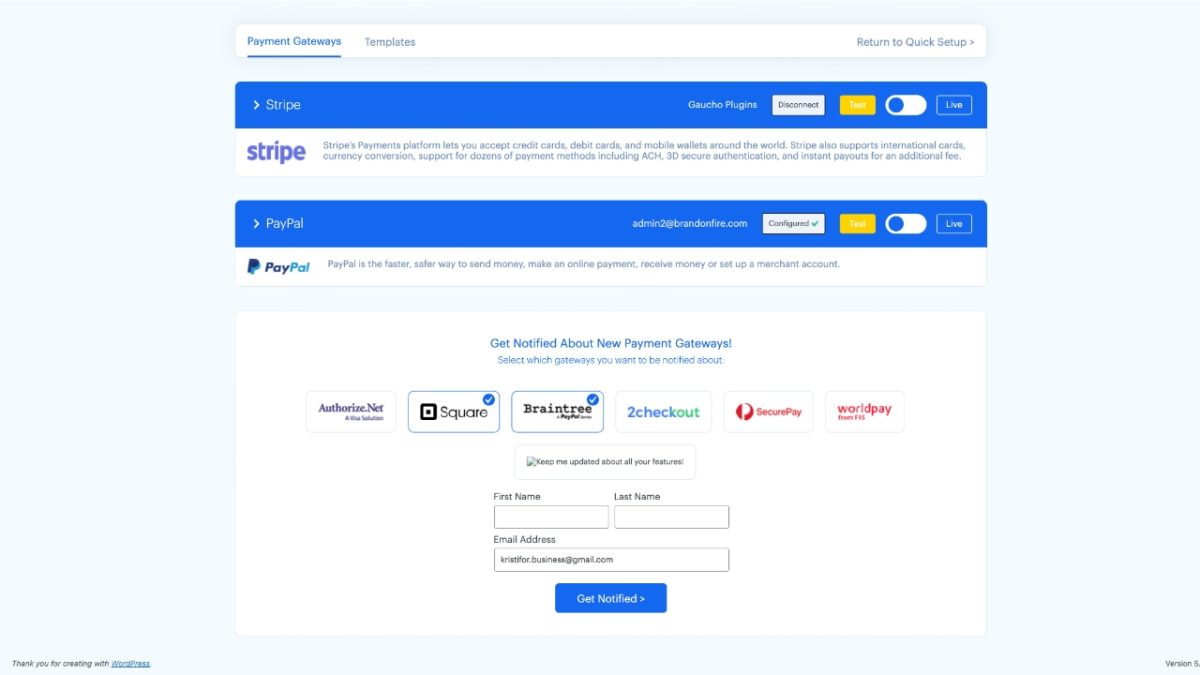Here is the cleaned-up and detailed caption for the image:

---

The screenshot captures the 'Payment Gateways' section within an application interface. At the top, a white header bar displays the text "Payment Gateways," with a link to "Return to Quick Setup" located on the far right.

Below the header, a long blue rectangle features the text "Stripe" prominently. To the right of "Stripe," there are options for "Disconnect" and a yellow rectangle labeled "Test." Adjacent to these, there is a toggle button allowing users to switch between "Test" and "Live" modes. Beneath this blue stripe, the word "Stripe" is displayed in large font, accompanied by additional details in very small print.

Further down, another blue rectangle labeled "PayPal" is present. Next to "PayPal," there is a person’s email address and the indication "Configured." Similar to the Stripe section, there is a yellow rectangle labeled "Test" and a toggle button for switching between "Test" and "Live."

Immediately following this is a white rectangle that reiterates "PayPal" and includes a brief description stating: "PayPal is the fastest, safer way to send money, make online payments, receive money, or set up a merchant account."

Below this description, there is a large white rectangle titled "Get notified about payment gateways." This section lists various payment gateways, including "Authorize.net," "Square," "Braintree," "2Checkout," "SecurePay," and "WorldPay."

At the bottom of this section, there are text boxes for entering "First Name," "Last Name," and "Email Address." Centrally located at the bottom of the screenshot is a button labeled "Get Notified."

---

This caption provides a thorough description of the various elements present in the screenshot, detailing their positions and functionalities.